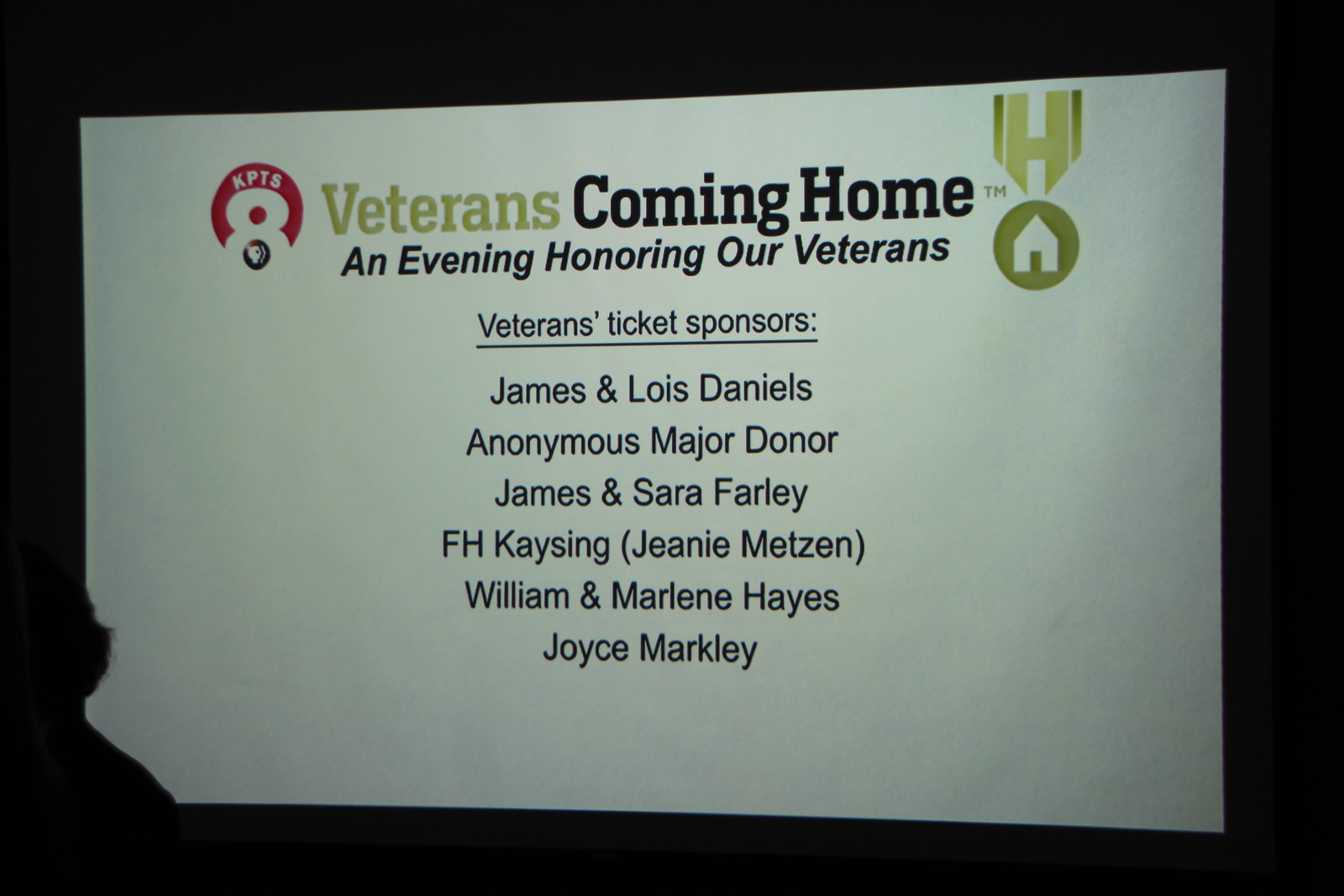This image is a presentation slide with a predominantly white background. In the upper left corner, there is a red circular logo featuring a white number "8" with "KPTS" written in white letters. The title of the slide, "Veterans Coming Home," is prominently displayed, with "Veterans" in green text and "Coming Home" in black. Below the title, italicized in black text, it reads "An Evening Honoring Our Veterans." To the right, there is a lime green ribbon lanyard featuring a green circle with a white house in the center. Beneath the main title, the section titled "Veterans Ticket Sponsors" is underlined, followed by the names: James and Lois Daniels, Anonymous Major Donor, James and Sarah Farley, F.H. Kaysing, Jean Metzen, William and Marlene Hayes, and Joyce Markley.